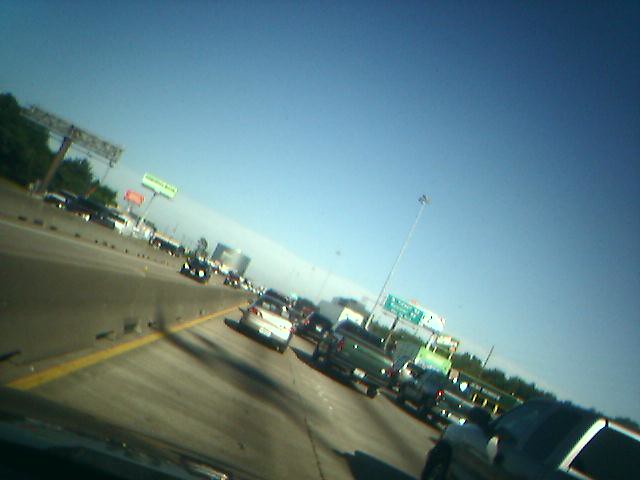This is a color photograph taken from a tilted angle, likely from inside a vehicle, capturing a busy highway scene. The image appears somewhat underexposed, possibly due to poor lighting or a low-resolution camera, and is tilted slightly to the right, nearly diagonal. The upper half of the photo features a blue sky with a low, flat layer of clouds on the horizon. 

We find ourselves in the left lane of a multi-lane highway, evidenced by multiple vehicles in the adjacent lanes to the right, including a grey truck and several other cars, indicating heavy traffic. The bottom left corner of the image shows a grey dashboard, reinforcing the perspective from inside a vehicle. To the left, there's a barrier separating oncoming traffic from the opposing direction, and some billboards, one red and one green. Dark trees are visible on both sides in the distance.

A green traffic sign with white writing is blurred to the right, hinting at upcoming exits. A series of tall street light poles extends into the distance. Additionally, there are two more traffic signs with yellow and red colors. In the far background, big containers and multiple lanes of traffic going in the opposite direction can be seen, separated by barriers.